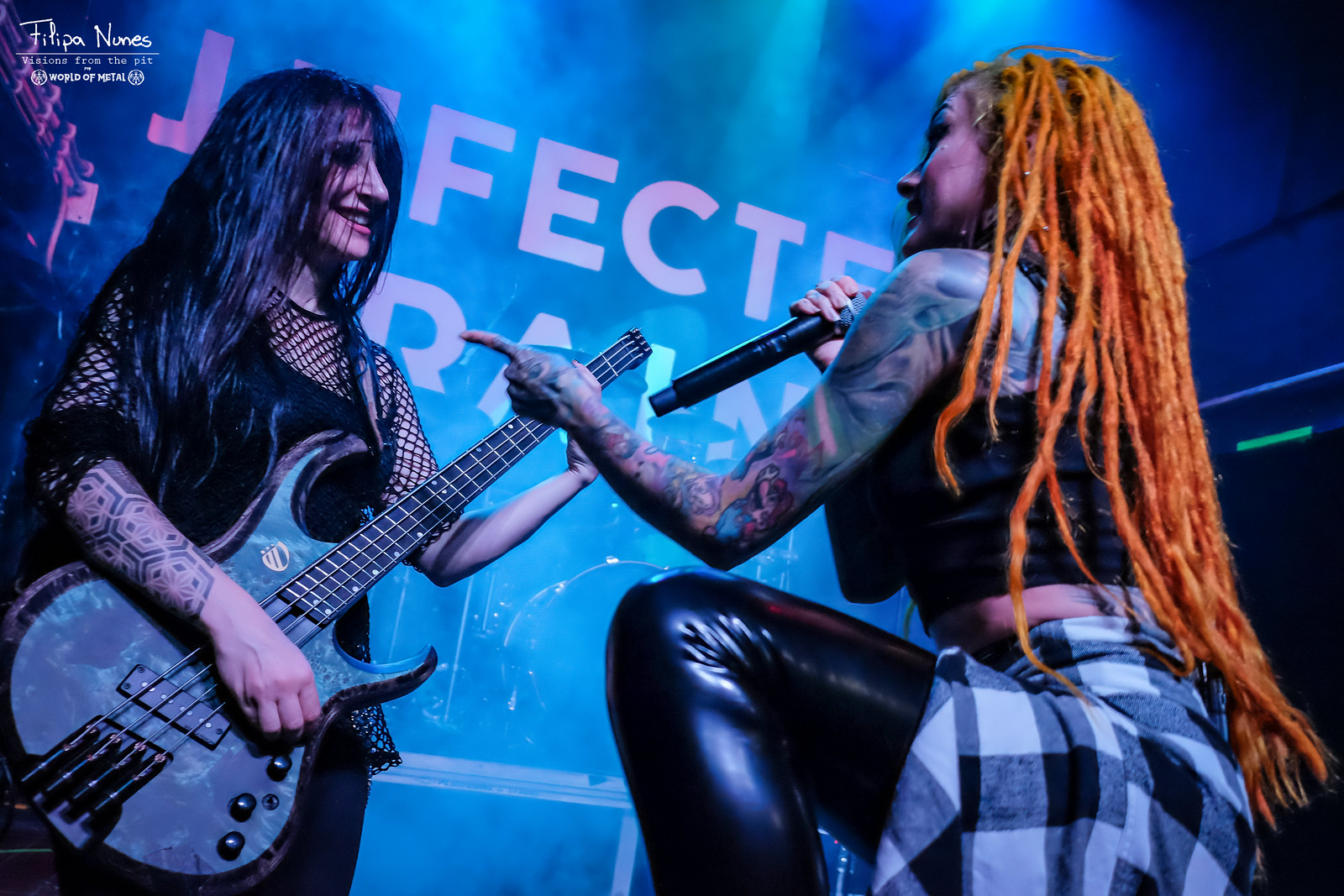The photograph captures an electrifying moment of a band in mid-performance on a shadowy, fog-laden stage. In the foreground, two female musicians dominate the scene. On the left, a woman with long black hair and colorful tattoo sleeves stands confidently holding a black electric guitar. She is dressed in a black tank top with fishnet sleeves. Opposite her, a woman with striking orange dreadlocks is captured in a side profile as she kneels down, gripping a microphone in her right hand. She sports a black crop top with skinny shoulder straps and a plaid skirt. Between them, elevated on a higher platform, sits a drum set, partially obscured by the swirling artificial smoke and fog projected onto a back wall. Although partially hidden, there is text on this back wall, adding to the atmospheric depth of the setting. Overhead spotlights punctuate the darkness, casting dramatic shadows around the room, highlighting the intense and raw energy typical of a rock concert.